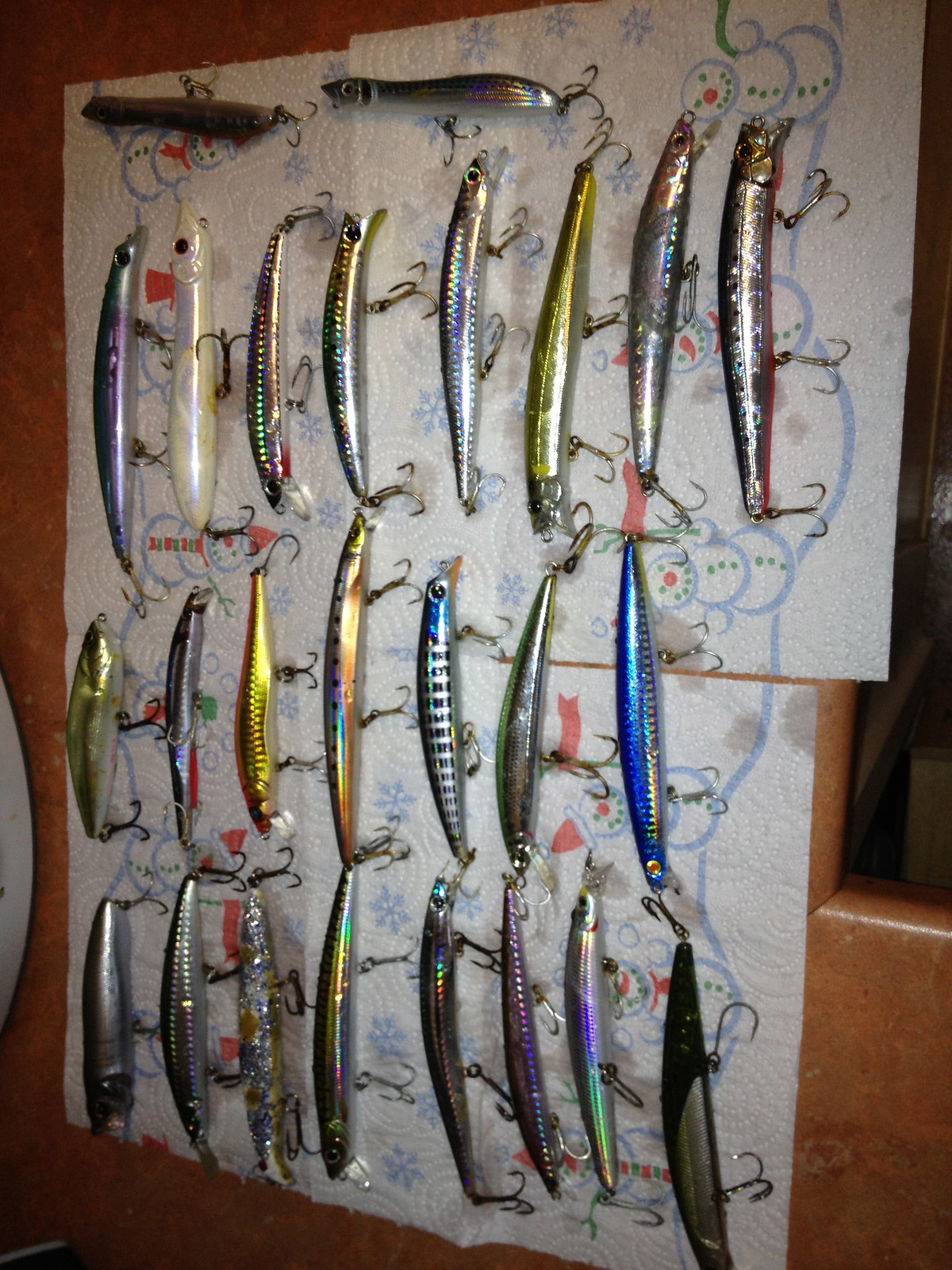This photograph features an intricately detailed setup against a brown wooden background, possibly a wall. Various fishing lures, crafted from metal and plastic, are arranged on paper towels. These paper towels are adorned with snowmen illustrations and are slightly damp, suggesting recent use or a water application. The lures themselves are diverse in both color and design, including hues like blue, orange, gold, silver, green, purple, and mixtures of yellow and orange. Each lure, resembling small fish, is equipped with multiple hooks and features details like black eyes and a sparkly, iridescent finish. Additionally, the lures are organized in three distinct rows on the paper towels, which also display small decorative elements akin to snowflakes. The entire collection is meticulously laid out, showcasing the variety and vibrancy of the lures against the festive, wintry paper backdrop.